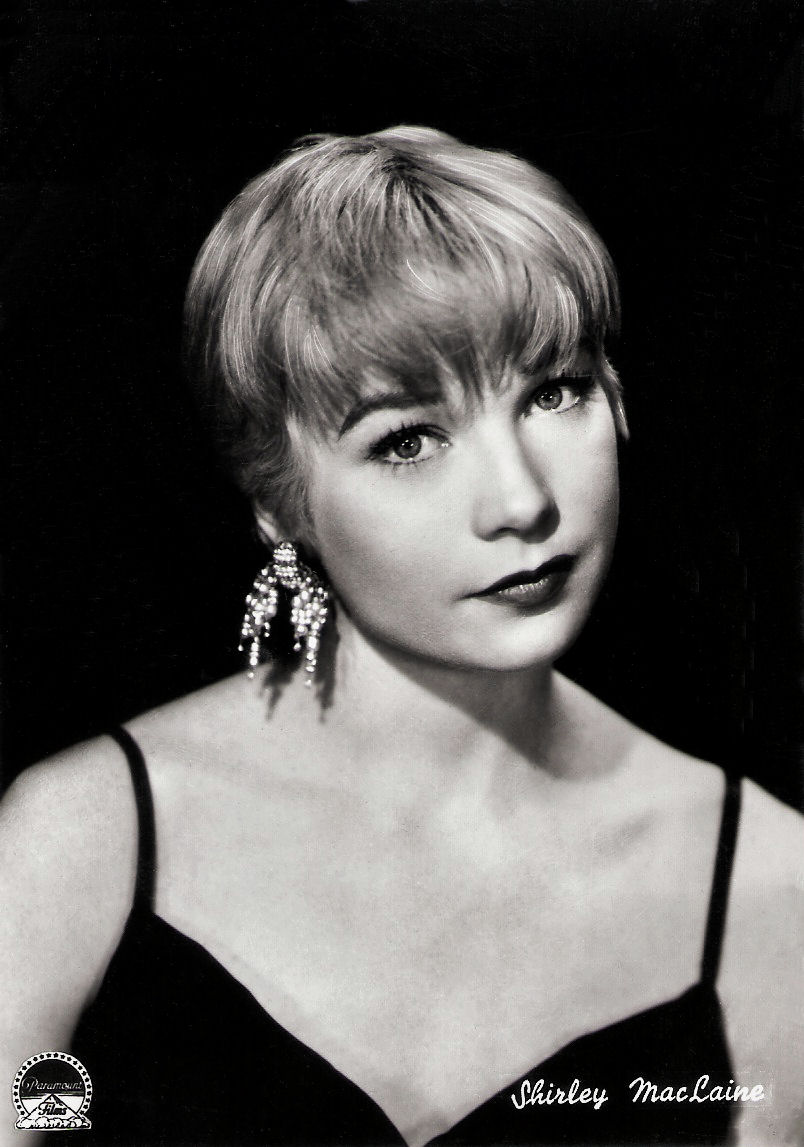This is a highly detailed black and white portrait of a young Shirley MacLaine, captured in a classic and elegant pose. The background is solid black, adding to the dramatic contrast of the image. Shirley is gazing directly into the lens with a neutral expression, her head slightly tilted. She is adorned with bold lipstick and exquisite dangling earrings that appear to be diamond-studded, adding a touch of glamour. Her hair is short, styled in a longish pixie cut that frames her face beautifully. She is dressed in a black dress with thin shoulder straps and a v-neckline, revealing her bare arms and chest, with no necklace to distract from her striking features. In the lower left corner of the image, there is a circular Paramount Films logo, while the lower right corner features her name, "Shirley MacLaine," elegantly written in cursive. Overall, the portrait exudes a timeless and sophisticated aura, likely taken in a professional indoor studio setting.